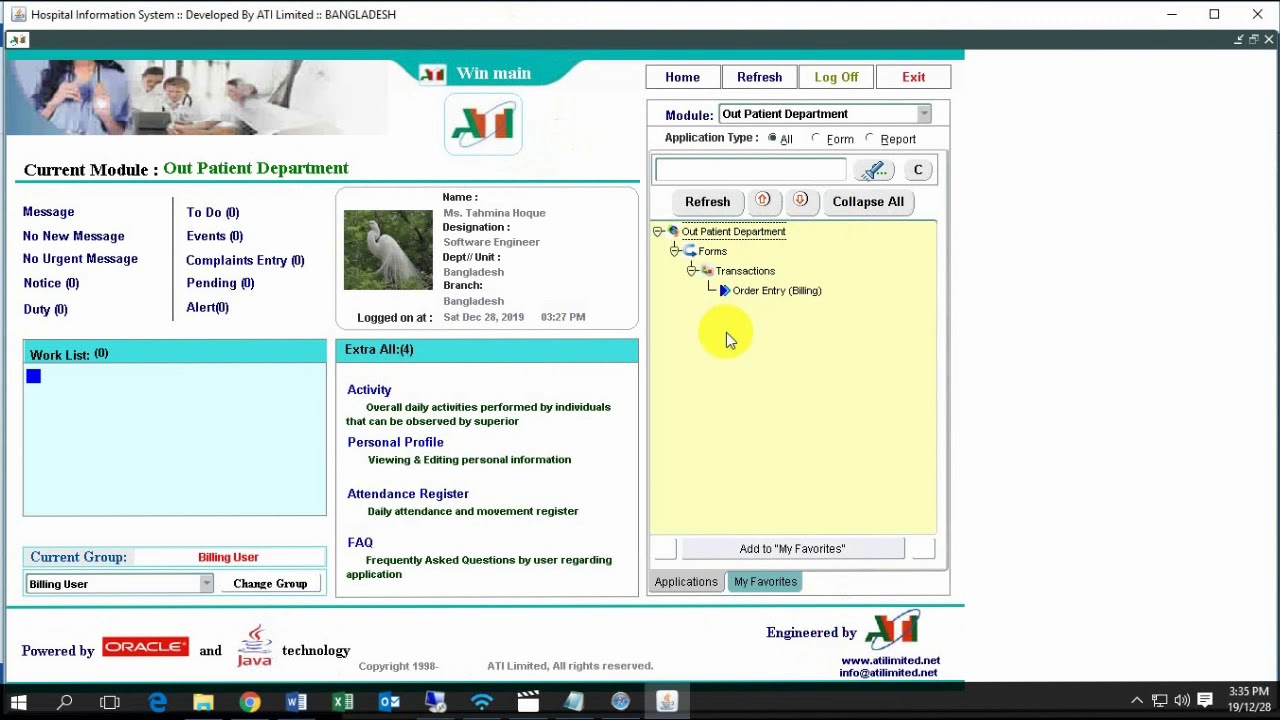This image depicts a web page from a hospital information system developed by AT Limited, Bangladesh. The page features a prominent green border at the top. Centrally displayed is an image of young residents, possibly medical trainees, engaged in studying; they appear to be examining a book or similar material. Among them, prominently visible on the left, is a young woman with long brown hair, wearing a stethoscope around her neck and holding it with both hands.

Additionally, the web page includes several sections and features. At the top, it displays "Current Modal" and various hospital department tabs like "Outpatient Department," which currently shows messages like "No message," "Duty," "Events," and "To Do." There is also a listing that seems specific to Bangladesh, indicated by a small icon of a bird.

Below these sections are some operational lists titled "Work List" and "Extra O List." To the right side of the page, there is a chat box with headings corresponding to different individuals. A yellow box, containing various sliding elements, and a yellow circle are also part of the layout, perhaps signifying notifications or alerts.